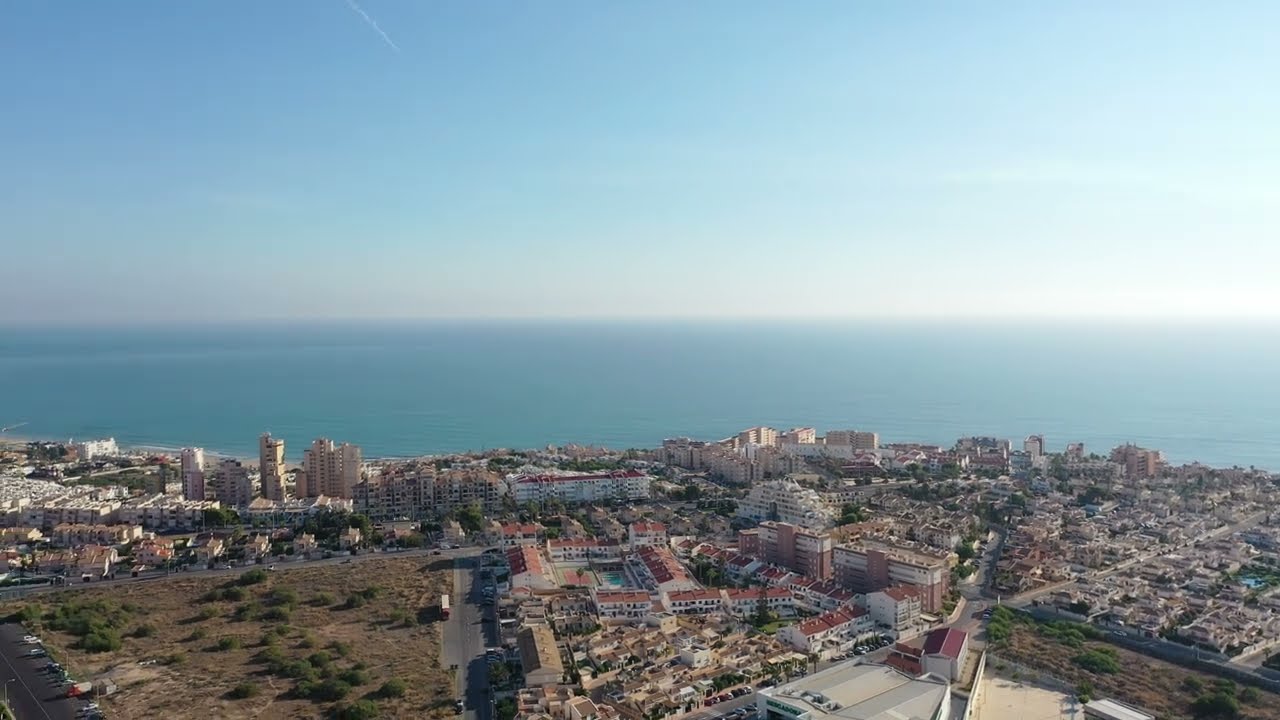This aerial view captures a picturesque city sprawling right to the edge of the ocean. Dominating the scene is the remarkable blend of residential and commercial zones, characterized by uniform, single-story houses and taller, more varied structures. A road carves its way from the city center, angling toward the right, guiding the eye to notable landmarks. Central to the image are buildings with distinctive white walls and sloped red roofs, adjacent to taller structures adorned with orange-colored walls, white sections at the top, and flat roofs. Behind these stand a white arch-like building and even further back, a strikingly tall edifice with white walls and a red-capped top. Toward the left, the cityscape transitions to taller, light brown buildings and an open expanse of vacant land dotted with brown brush and green bushes. The city's vibrant activity extends from the left to the right, with an endless succession of buildings. In the distance, the serene, light-blue ocean meets a bright, mostly clear sky with hints of haze and a strikingly bright white light on the right. This image, possibly captured by a drone or aircraft, vividly portrays a harmonious blend of urban life and natural beauty.